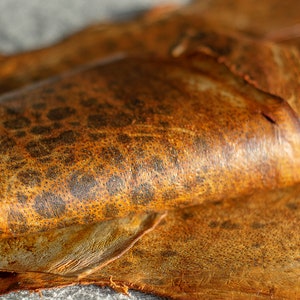This highly-cropped, square photographic close-up appears to show treated animal skin or leather. The piece, light brown with dark brown spots and a shiny, reflective surface, is folded or shaded in a manner that almost resembles a holster. It is positioned on another, similar flat piece of leather, also light brown with dark brown spots. At the bottom of the image, a gray and white textured tablecloth is partially visible. The top corners of the image are out of focus, with the gray tablecloth discernible in the top left corner. The overall image is sharply focused in the foreground, gradually becoming blurred towards the background, and devoid of any identifying text or other clues.